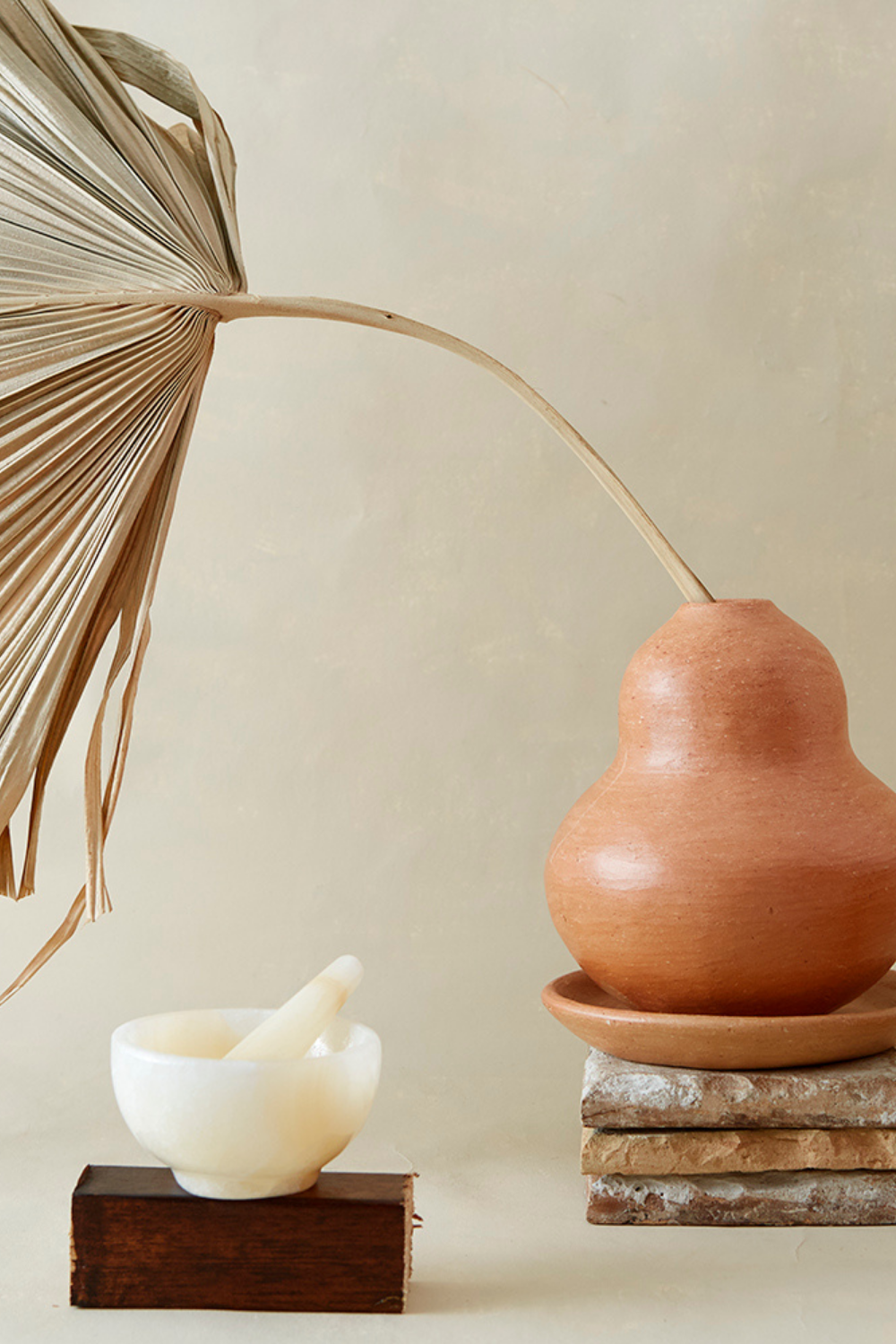The image displays a modern still life featuring a large, gourd-shaped vase in an orangish-brown hue, reminiscent of terracotta pottery. This simple yet striking vase, which appears to have been handmade on a pottery wheel, is seated on a matching round plant plate. A single, large, dried brown palm frond extends from the top of the vase, leaning gracefully to the left. The entire arrangement is set on three perfectly stacked stone tiles, with the top and bottom tiles in a grayish-white shade and the middle one in a terracotta color.

In the foreground, to the left, a brown wooden block, rough-cut and slightly splintered, supports a creamy white marble mortar and pestle set, adding an additional layer of texture to the composition. The background contrasts in ivory tones, enhancing the earthy colors and natural materials in the foreground, creating a serene, harmonious scene.